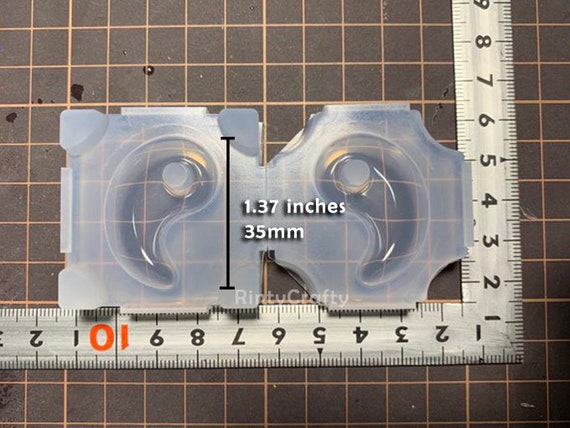In this photograph, a white semi-transparent plastic product is prominently featured on a dark brown surface, which is adorned with a grid of light brown lines forming small squares. Central to the image is the plastic item, characterized by two drop-like depressions and an asymmetrical shape—square on the left and octagonal on the right. This product has been annotated with a black vertical line and white text indicating its dimensions: "1.37 inches" and "35 mm." Below this plastic product lies a metallic L-shaped ruler. The ruler has measurement markings in inches, numbered 1 through 4, written in black, with the number 10 in red. The ruler's orientation allows it to measure both horizontally and vertically, aligning with the grid pattern on the surface, which resembles that of a self-healing cutting mat or metric paper.